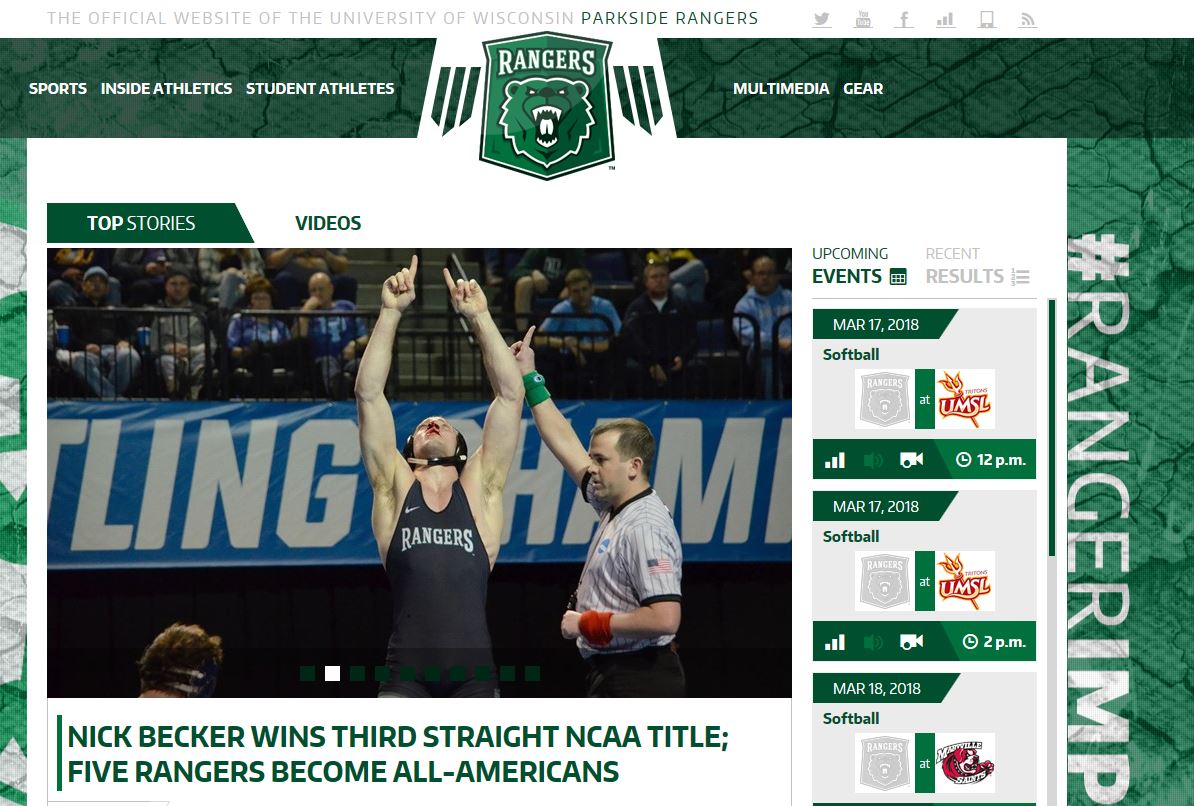The official website of the University of Wisconsin Parkside Rangers' athletic department prominently features the university's green and white color scheme. At the top, the website displays "University of Wisconsin Parkside Rangers" in a light-colored font, accompanied by the Rangers logo, which appears to be a bear. A dark green navigation bar spans the top, offering drop-down menus with white font that allow visitors to explore different sports, behind-the-scenes content, student-athlete information, multimedia resources, and available merchandise.

The main body of the website is divided into two sections. On the left, a "Top Stories" tab is highlighted by a large image of a victorious wrestler, showcasing recent achievements. On the right, there is a schedule of upcoming events, specifically focusing on various softball games that are about to commence. The layout clearly organizes the latest news and important dates, providing a comprehensive overview of the university's athletic activities.